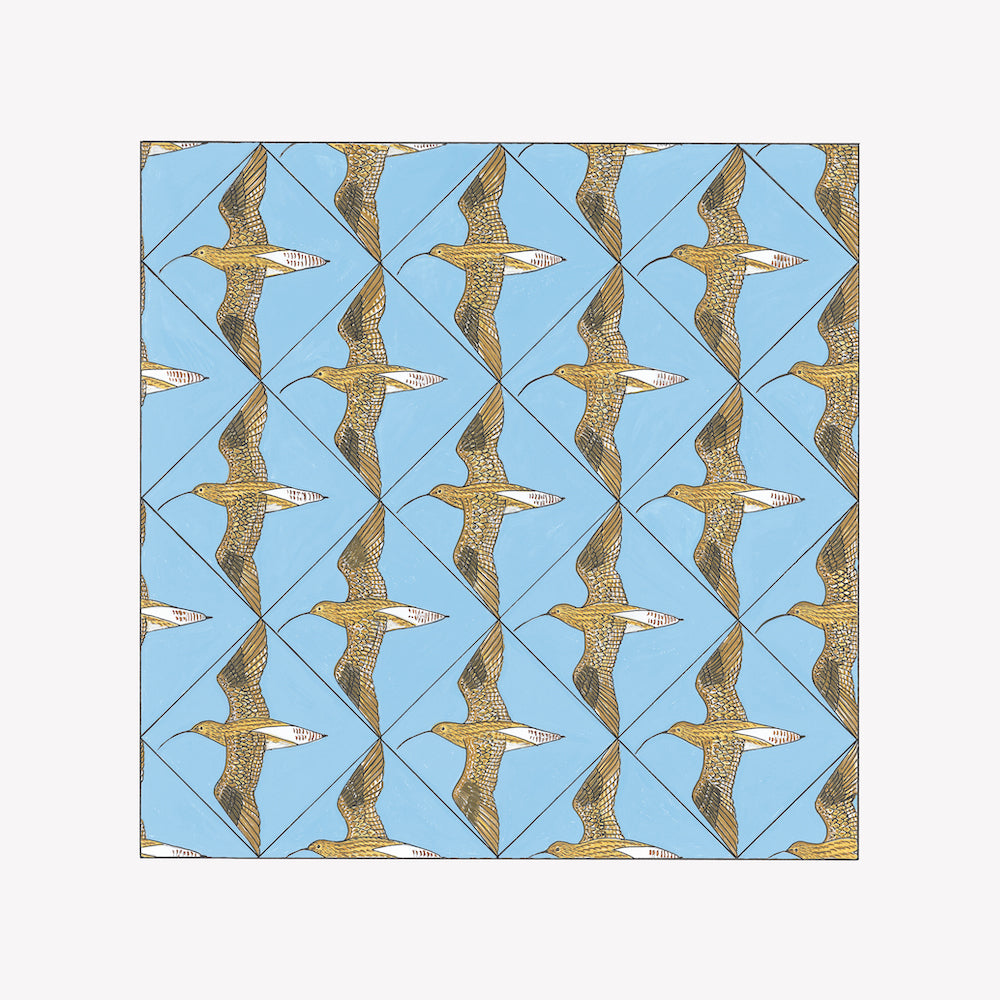This intricate artwork features a repetitive pattern of gold and brown hummingbirds set against a rich teal blue background. Each bird is positioned within diamond-shaped grids formed by bold black lines. The hummingbirds are depicted with wings fully spread, showcasing a mix of gold, white, and brown hues, while their long, curved black beaks and tiny black eyes add detail to the composition. The wings and elongated beaks often extend beyond the confines of the diamonds, particularly at the edges of the image where only parts of the birds are visible. The diamond pattern continues uniformly across the vertical artwork, with 13 complete diamonds and 8 partial ones, creating a rhythmic tiled effect that spans the entire design.